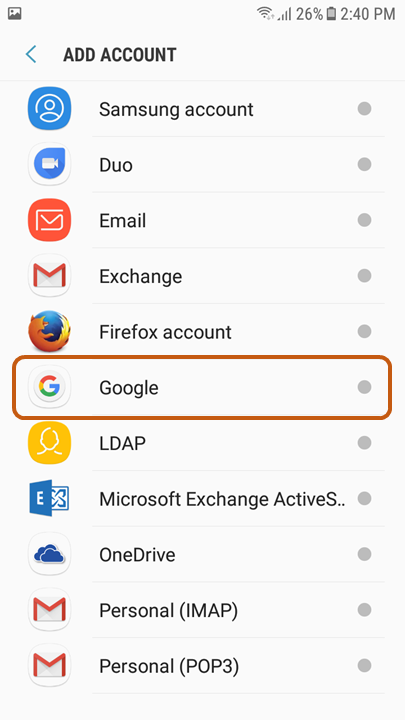This image captures a cell phone settings submenu specifically for adding accounts. In the upper right-hand corner of the screen, icons indicate the status of the phone: a Wi-Fi symbol, cellular signal bars, and a battery icon showing a 26% charge. The time displayed is 2:40 PM. The submenu presents a variety of account types available for selection, listed from top to bottom as follows: Samsung account, Duo, Email, Exchange, and Firefox. The "Google" option is highlighted in the image. Following Google, the list continues with LDAP, Microsoft Exchange ActiveSync (indicated with ellipses suggesting that part of the text is cut off), OneDrive, Personal IMAP, and finally, Personal POP3.